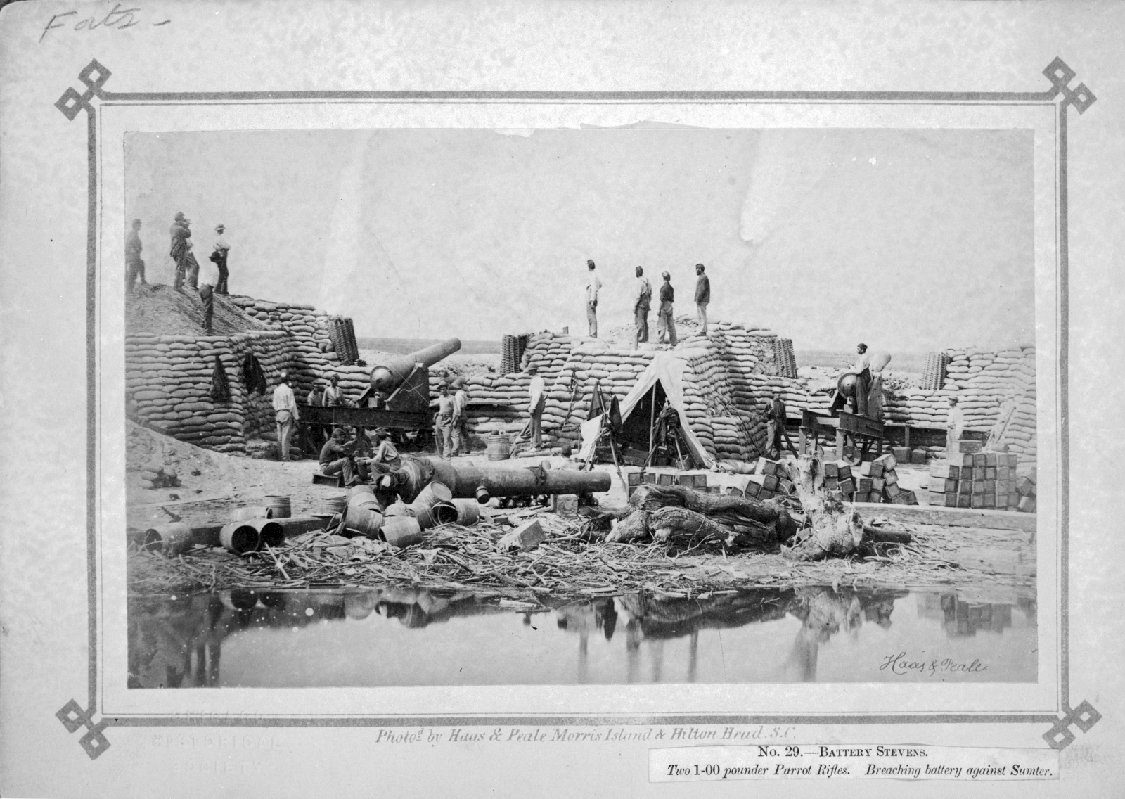This image is an old, black and white photograph, centrally positioned on a piece of gray paper. The photograph, likely taken in the late 1800s or early 1900s, depicts a military bunker or fortification. The primary structure consists of many sacks of sand or soil, carefully stacked to form protective earthenworks. Atop these embankments stand several men, dressed in period-appropriate attire, indicative of a military setting, possibly discussing their duties or overseeing operations. Prominently featured are large cannons—one visible on the top of the structure pointing towards a large body of water in the background, and another cannon lying in the foreground beside a small swampy water body. The bottom right corner of the photograph bears an inscription, though partially illegible, suggesting historical context with terms like 'Battery Stevens' and '2100 Pounder Parrot Rifles.' Additional text beneath the photograph on the gray paper may read: "No. 29 Battery Stevens 2100 Pounder Parrot Rifles Breaching Battery Against Sinter," adding further detail about the military equipment and potentially the location or purpose of the battery.